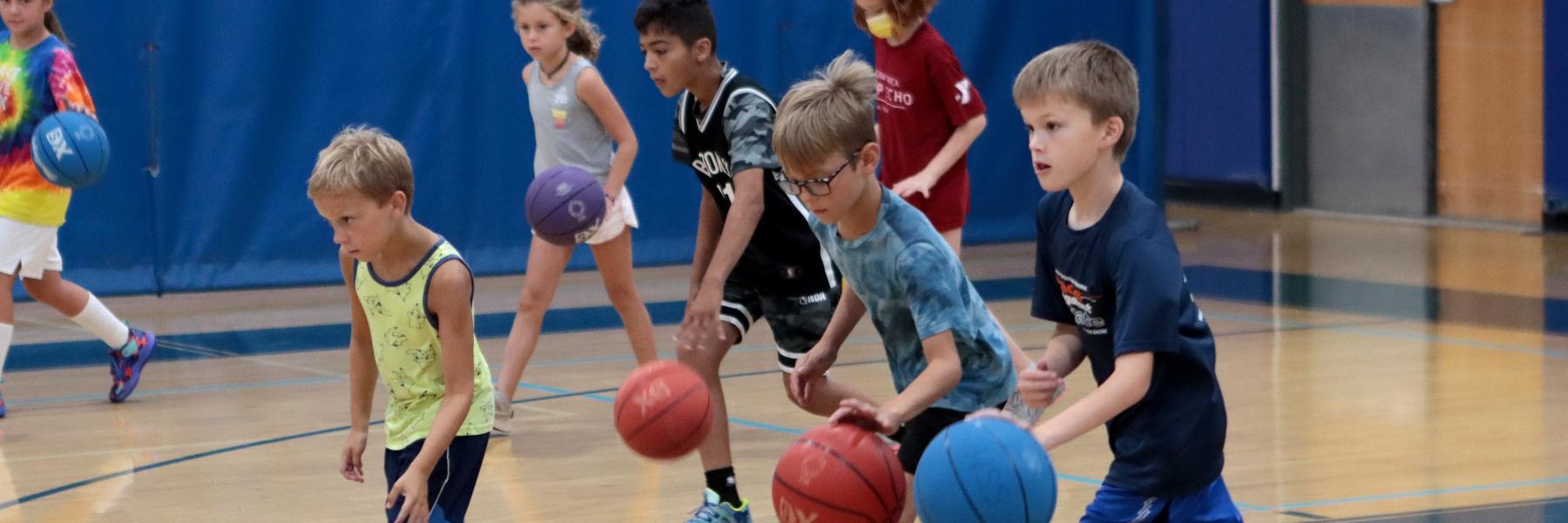This image captures a lively scene set from the sidelines of a school gymnasium, featuring seven children—an equal mix of boys and girls, aged approximately 5 to 10 years old—actively practicing their dribbling skills on a typical brown basketball court outlined in blue. The children, belonging to diverse ethnic backgrounds, including Caucasian and brown, are dressed in a variety of colorful shirts and shorts. Each child is seen concentrating intently as they dribble basketballs in a harmonious rhythm. The basketballs themselves are vividly colored in blue, red, and purple hues. A notable background detail includes a kid wearing a yellow mask and a red shirt, standing out against the blue wall and curtain framing the scene. The atmosphere is energetic and focused, highlighting the children's dedication and enjoyment of the sport.